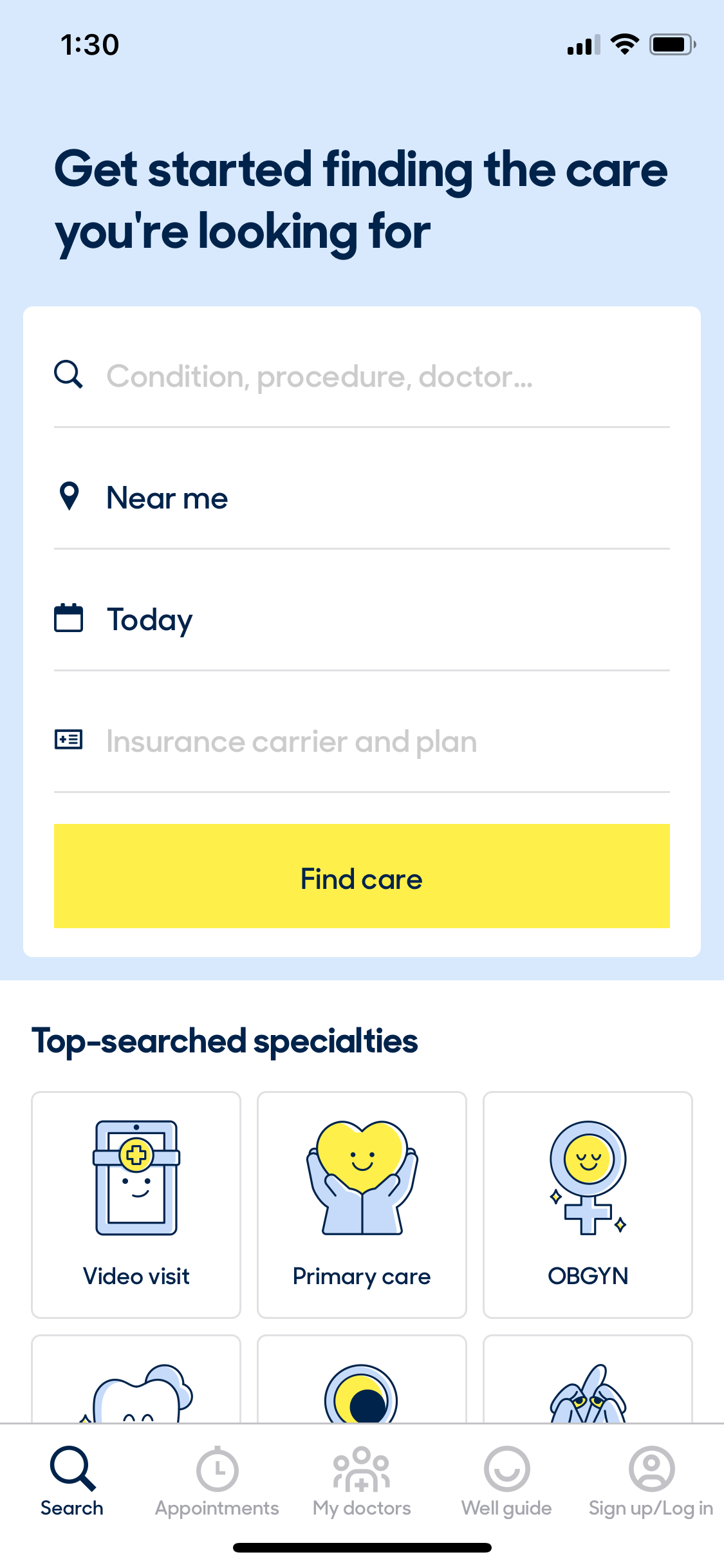**Detailed Caption:**
This image is a screenshot taken from a tablet or smartphone interface. 

**Top Bar Details:**
- The left side of the top bar displays the time as 1:30, without specifying AM or PM, hinting at the possibility of military time settings.
- On the right side, the signal strength is shown as 3 out of 4 bars, while the Wi-Fi signal is full and the battery is almost fully charged with only a small portion missing. All these notifications are in black.

**Main Background and Text:**
- The main background is cyan blue.
- Bold black text in the center reads: "Get started finding the care you are looking for."

**Search Interface:**
- Below this text, there is a white rectangle divided into different sections by grey lines:
   - **First Section:** Contains a black magnifying glass icon and the grey text "condition, procedure, doctor…" followed by a black pen-like icon and the text "near me" in black.
   - **Second Section:** Depicts a calendar icon with the text "today".
   - **Third Section:** Features an icon resembling a piece of paper with three horizontal lines on the right, a plus sign on the left, and the grey text "insurance carrier and plan".

- Beneath these sections, there is a yellow button with the black text "Find care" centered in it.

**Specialties Icons:**
- Below the button, the text "Top-searched specialties" is displayed.
- Various buttons in square shapes depict different specialties:
   - **Video Visit:** A blue-outlined square with a yellow circle containing a plus sign, two eyes, and a mouth.
   - **Primary Care:** An icon resembling a blue doctor's vest with a yellow heart, two eyes, a smiley face, and arms raised.
   - **OBGYN:** A medical cross with a yellow face, closed eyes, a smile, and two diamond shapes on either side.
   - **Dental Care:** A tooth icon next to a partially cut-off cyan blue circular object that transitions to yellow and dark blue towards the center.
   - **Additional Icons:** At the bottom-right, there appears to be a slightly droopy character with a pointy head and droopy sides, also partially cut off.

**Bottom Navigation Bar:**
- The bottom bezel contains various navigation options:
   - A black-highlighted "Search" option.
   - A faded stopwatch icon labeled "Appointments".
   - Silhouettes of people, indicating "My doctors".
   - A circle with a semicircle inside it labeled "Well guide".
   - An icon of a circle for the head and a semicircle for the body indicating "Sign in, access, log in" in grey.
- Below these icons, an oval bezel is visible for general navigation and exiting out of the interface.

This descriptive caption provides a comprehensive overview of the screenshot content for better understanding and accessibility.